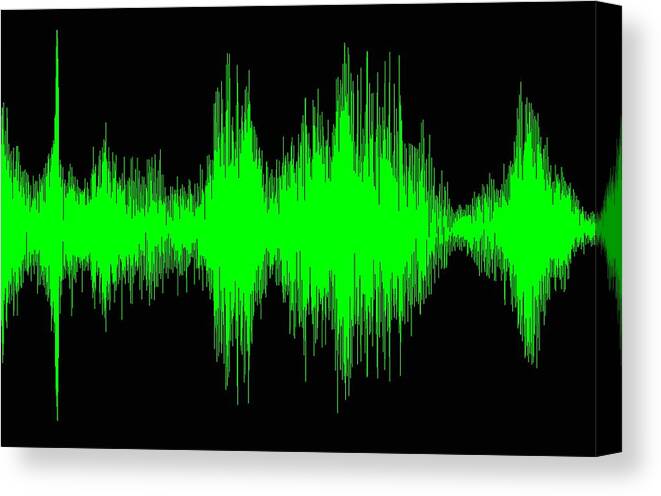The image features a three-dimensional black rectangular canvas displaying a vivid lime green representation of sound waves. These waves, indicative of a high-pitched sound, fluctuate in height and density as they traverse from the left to the right side of the canvas. Initially, the waves are closely bunched together, gradually increasing in height towards the center, which appears to be the peak of the high pitch. Following this central peak, the waves decrease in height somewhat, creating a dynamic, irregular pattern. The intricate detail of the waves, combined with the stark contrast of the green on black, lends the image a visually striking and complex appearance. The image could be interpreted as an oscilloscope trace or a recording visualized by a voice recording app, emphasizing the erratic nature of the sound depicted.